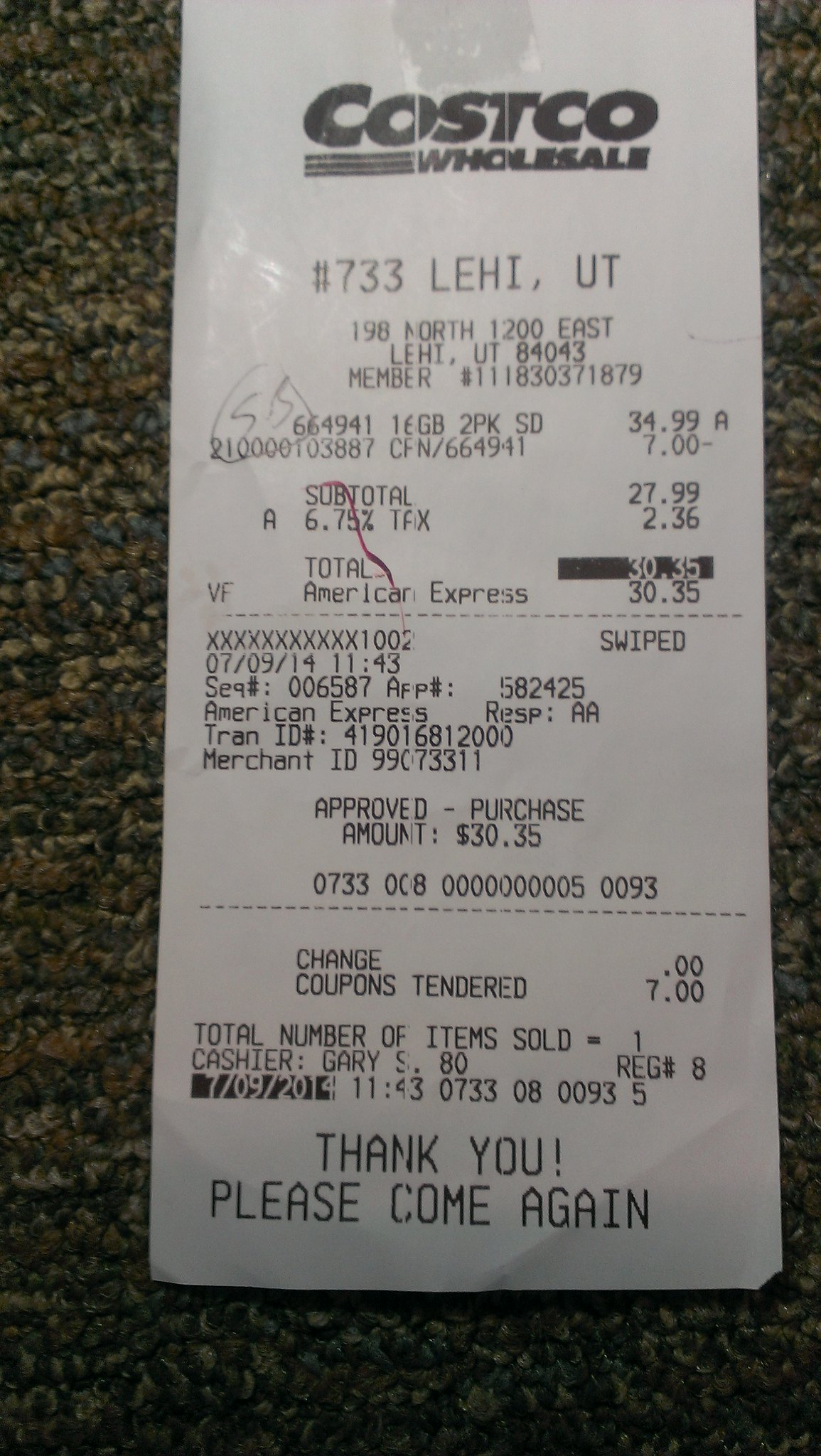A detailed, cleaned-up caption for the image could be:

"This image shows a Costco receipt laid flat on a green and cream-colored surface, likely a carpet. The receipt, from Costco Wholesale store number 733 in Lehi, Utah, details a transaction where the buyer received a $7 discount on an item, resulting in a total cost of $30.35 after tax. Payment was made using an American Express card. Towards the bottom, the receipt displays a polite thank you message, 'Thank you, please come again.' Additionally, the member number is clearly visible on the receipt."